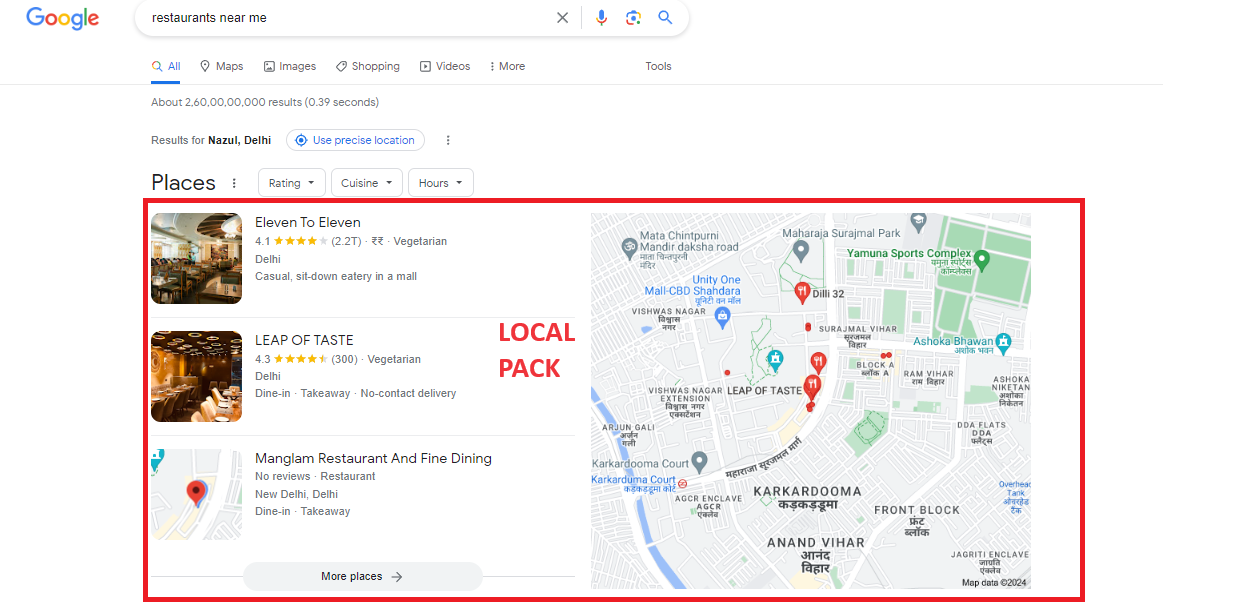This image shows a Google search results page for "restaurants near me" in Delhi, India. The interface is sleek and user-friendly, displaying over 2 billion results in under a second. The search results feature a list of restaurants accompanied by various interactive elements to refine your search.

At the top, three dropdown boxes allow users to filter results by rating, cuisine, and hours. You can select higher-rated places, choose specific cuisines like Indian or Italian, and filter by open hours.

The list of restaurant results includes detailed mini-profiles:
1. **11 11 Restaurant**:
   - Rating: 4.1 out of 5 stars
   - Price: Moderate (indicated by two emoji markers)
   - Cuisine: Vegetarian
   - Type: Casual sit-down
   - Image: Provided

2. **Leap of Taste**:
   - Rating: 4.3 out of 5 stars
   - Price: Moderate
   - Cuisine: Vegetarian
   - Options: Dine-in, takeout, no contact delivery
   - Designation: Local pack
   - Image: Provided

3. **Maglum Restaurant and Fine Dining**:
   - Rating: No reviews yet
   - Cuisine: Fine dining
   - Options: Dine-in, takeaway
   - Image: Not provided

The right side of the image features a map with red pins, each marked with a fork and knife icon, indicating restaurant locations clustered along a similar route. Additional restaurant options are listed below these primary results for further exploration.